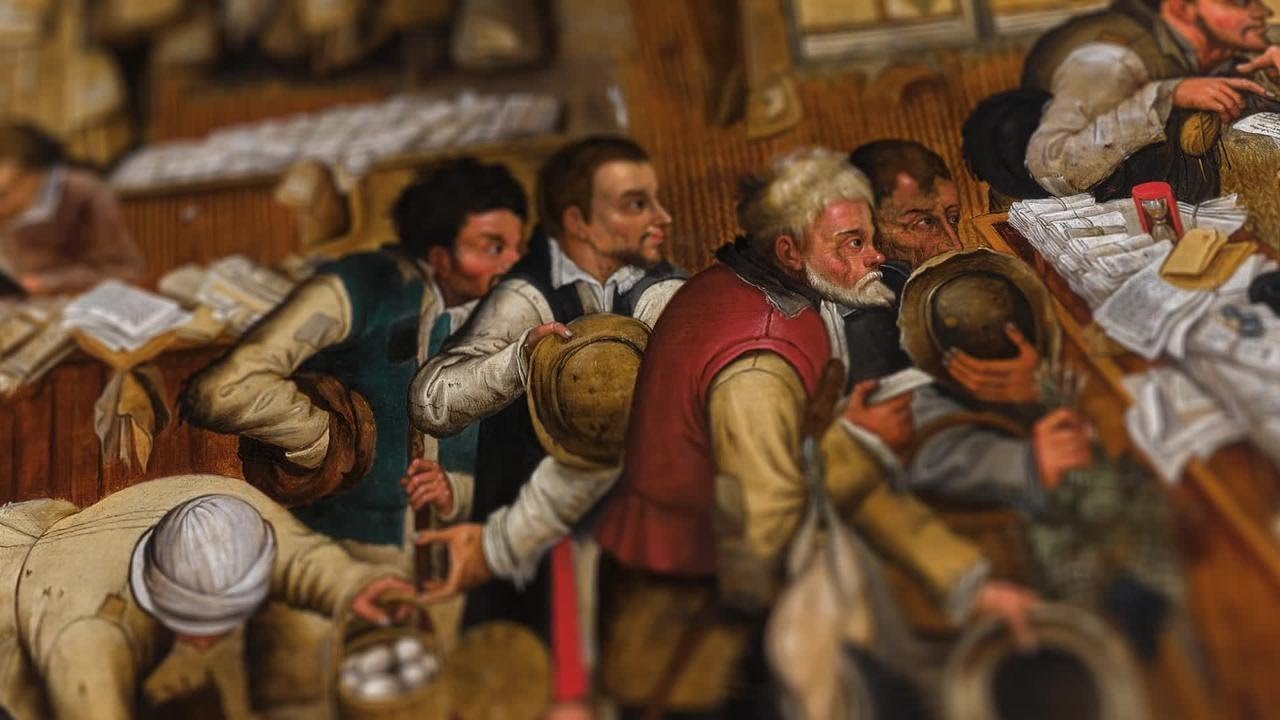The image is a detailed painting or colored illustration depicting a group of men in a room, possibly gathered around a bar-like wooden table or counter that extends from the bottom right to the left. There are stacks of white papers scattered or neatly arranged on this table. Prominently on the table, an hourglass with a red casing can be seen. 

In the foreground, several men are queuing up, each holding a hat in hand. Four men are standing in line in front of the table:
- The first man on the left is turned slightly and has his back towards the viewer, obscuring his full face with a hat. 
- Right next to him is an elderly man with white hair and a white beard, dressed in a striking red vest with white sleeves, and he appears focused towards the right.
- Behind the man in red stands another figure with short brown hair and a beard, dressed in black and white attire.
- The fourth man in the queue has somewhat long, black hair and is dressed in green and white apparel.

Additionally, there is another man beside the last man in the queue, either picking up something or falling forward. He is dressed in a slightly darker shade of white apparel than his white hat and leans towards the bottom left of the image.

In the far background, another wooden table with more papers can be seen, with a man sitting at it on the left side of the image. The upper left and bottom right corners of the image are somewhat blurry, adding a peculiar photographic effect to the illustration. A few other men are visible, their figures and actions partially blurred, giving the scene a sense of depth and activity. The setting, composed of wooden elements and scattered papers, imbues the painting with a historical or bureaucratic atmosphere.